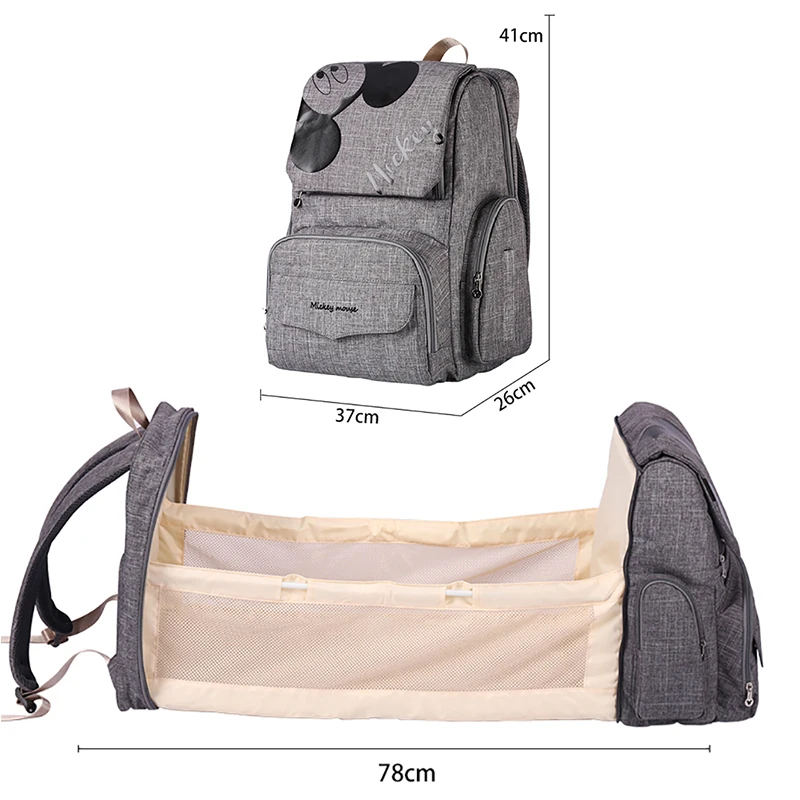The image showcases a versatile charcoal gray diaper backpack adorned with an upside-down image of Mickey Mouse's face on the top part, prominently featuring his black ears and eyes. The backpack has several practical compartments, including a top pocket, a front pocket, and a side pocket. The name "Mickey" is subtly embedded into the design. The backpack measures 37 centimeters in width, 26 centimeters in depth, and 41 centimeters in height. Notably, an expandable section at the bottom transforms into a beige, elongated rectangular changing bed for children, which extends to 78 centimeters wide. The image also delineates these dimensions and features, emphasizing the backpack's multifunctional use.